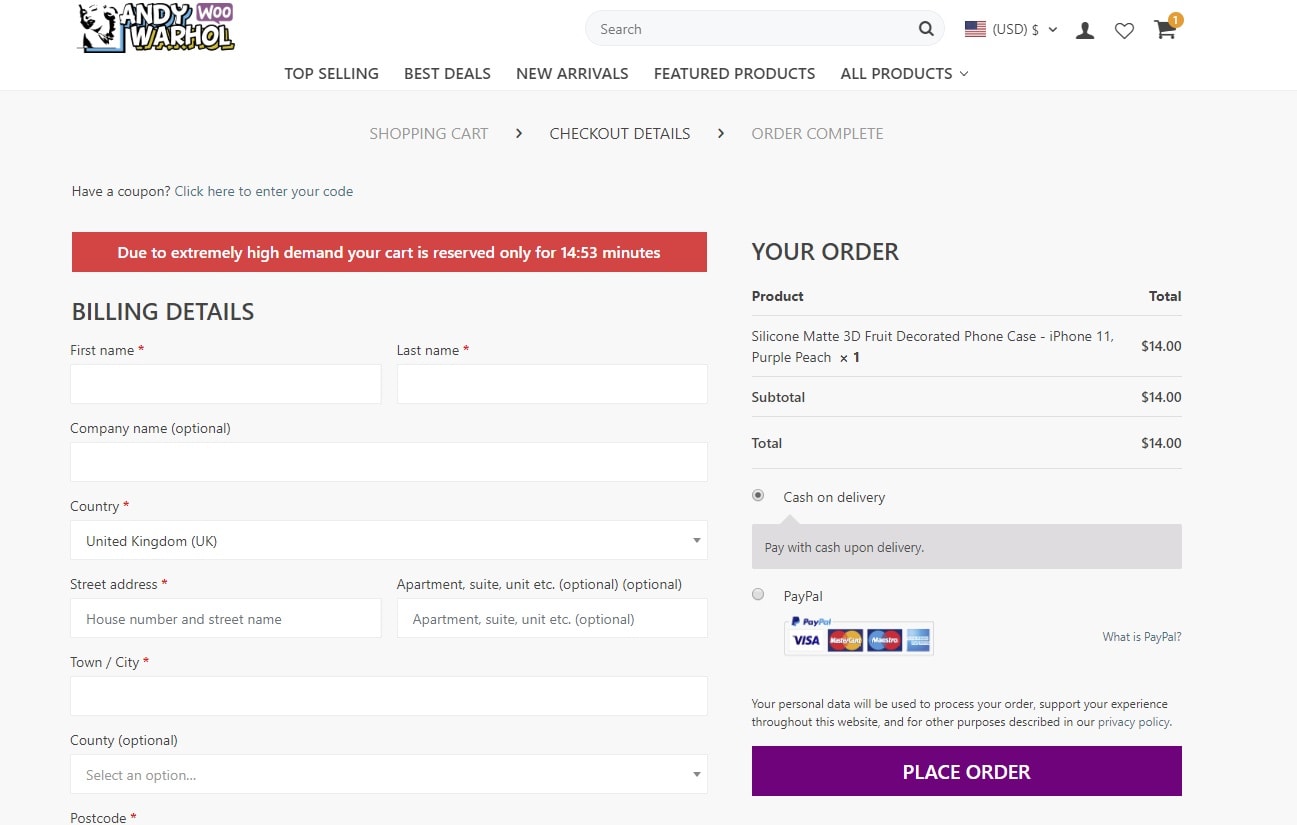The image is a screenshot from a website branded as "Andy Wu Warhol" at the top. On the top left of the site, there's a black and white image of a woman who closely resembles Marilyn Monroe. The top navigation bar features several dropdown options labeled "Top Selling," "Best Deals," "New Arrivals," "Featured Products," and "All Products." There is also a search bar with a magnifying glass icon, an American flag alongside "USD" indicating currency, and icons representing a human silhouette, a heart for wishlist, and a shopping cart with a yellow circle displaying the number one, indicating an item in the cart.

Scrolling down, the website outlines the shopping process with headings: "Shopping Cart," "Checkout Details," and "Order Complete." A blue hyperlink text prompts users with "Have a coupon? Click here to enter your code." Additionally, a prominent long, skinny rectangle warns visitors that "Due to extremely high demand, your cart is reserved for only 14:53 minutes." The webpage also includes fields for entering billing details and order information. At the bottom right corner, a striking purple button labeled "Place Your Order" is situated.